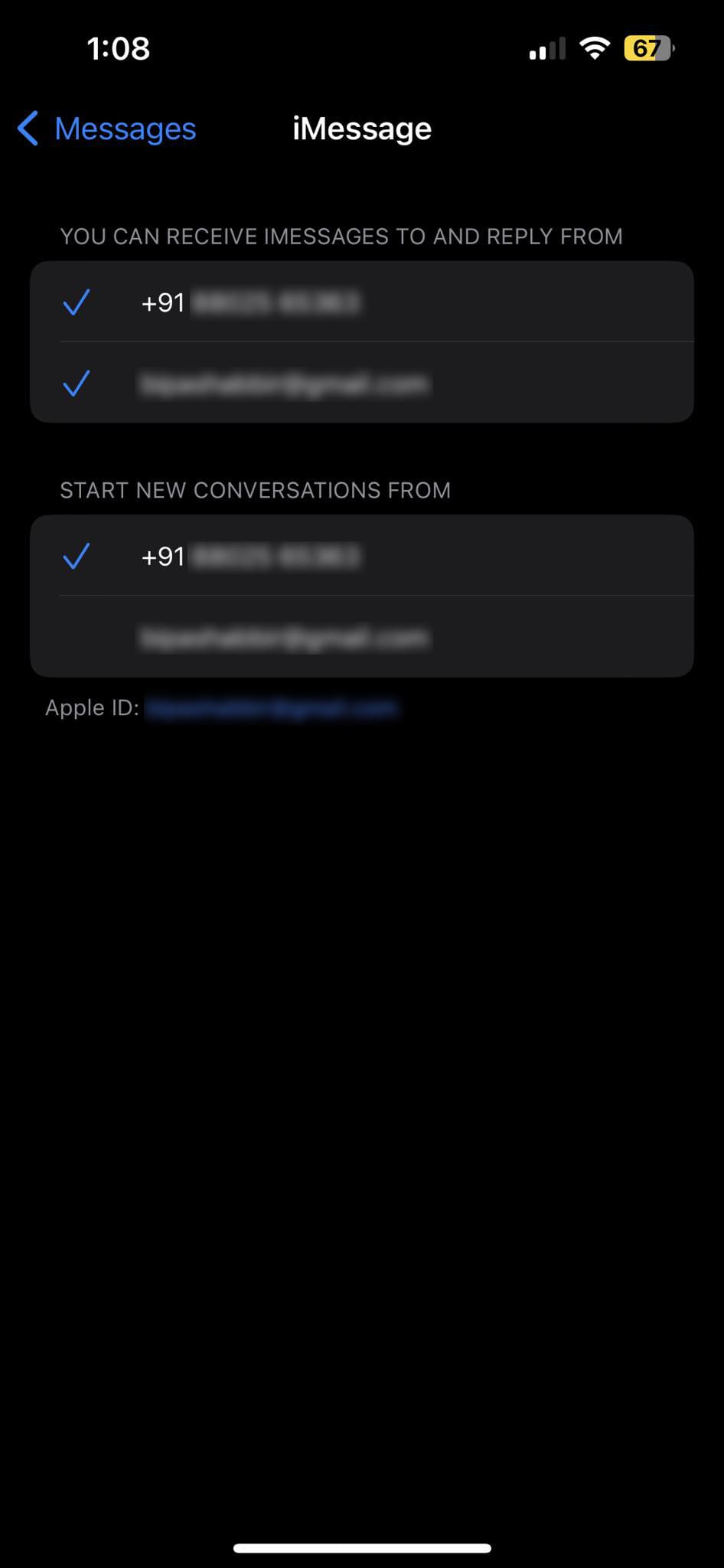The image depicts an iPhone screen in dark mode, specifically within the iMessage settings. The screen shows options to allow users to send and receive messages from a phone number and an email address, both of which are blurred but remain semi-visible in white and blue text, respectively. The Apple ID is also blurred out using a semi-transparent, fuzzy gauze effect. Additional screen details include a black background, a status bar indicating 67% battery life, a strong Wi-Fi connection, mediocre cellular signal, and the time displayed as 1:08. The rest of the screen and settings remain largely non-descript due to the dark mode background, offering minimal additional information.